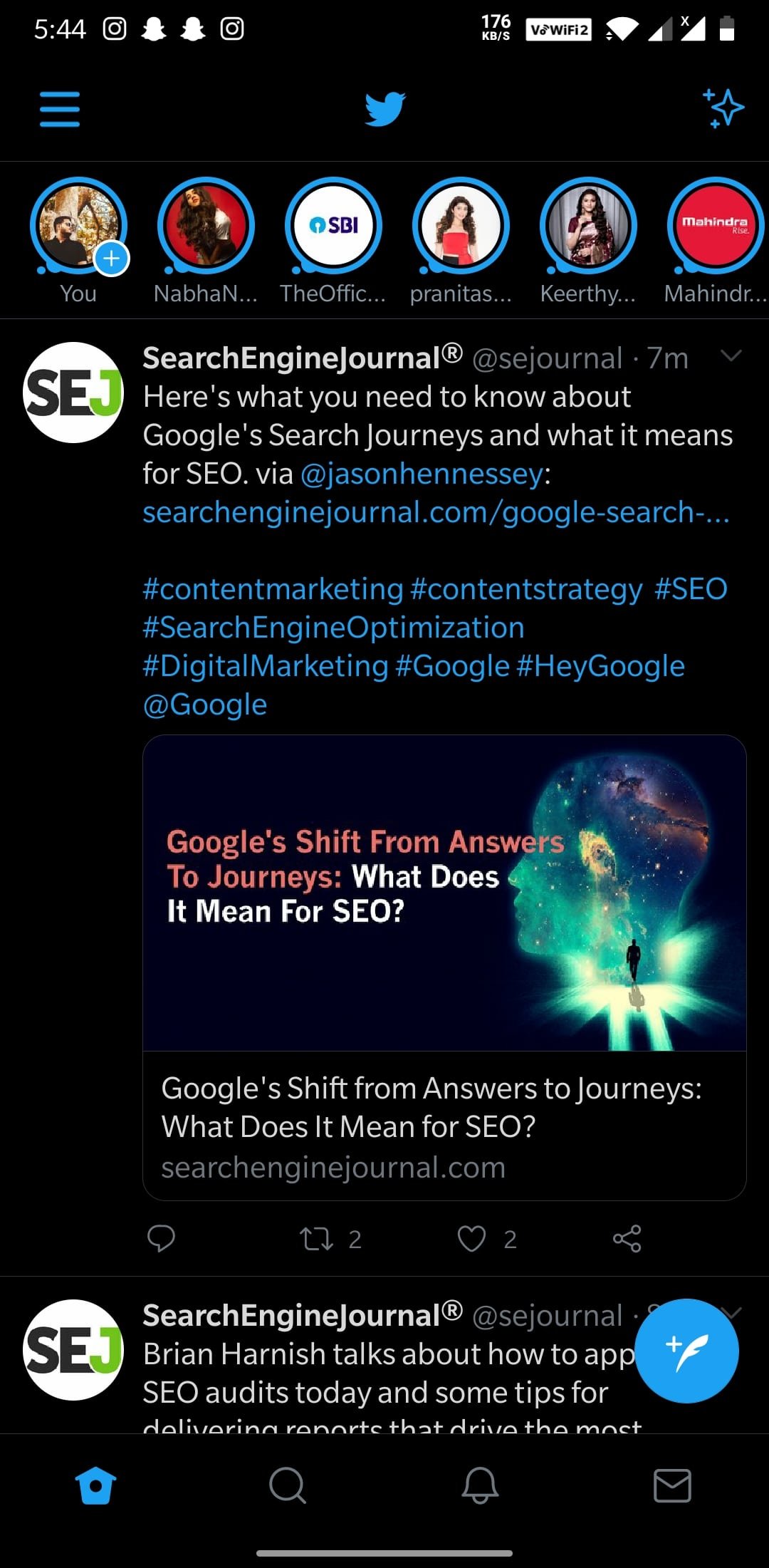A screenshot from a smartphone displays a variety of visual elements and icons characteristic of a typical social media post. 

In the top left corner, the time is set to 5:44. Adjacent to this is a sequence of four icons: Instagram (a square with a circle in the middle), two Snapchat ghosts, and another Instagram icon, followed by text showing "176" with some small, indistinguishable lettering below. Next is a small white rectangular box with unreadable characters, followed by an upside-down triangle with a rounded top, possibly indicative of some form of power measurement. To the right, three half-filled battery indicators are displayed, signifying battery life, alongside three blue signal bars that likely represent signal strength.

At the top center, a blue bird icon represents Twitter. The top-right corner displays two stars alongside a blue diamond, though their significance remains unclear. Below this is a series of circular images. The first two circles show pictures of women, followed by a white circle with a blue plus sign and the word "You" in white text. Adjacent are more images and logos: "SBI" in a blue circle, two more images of women with varying backgrounds, and another logo on a red background with white lettering.

Beneath the images are text descriptions: "You," followed by fragmented names and titles truncated with ellipses, such as "NABHA," "OFFIC," "Prentice," "Keerthy," and "MAHINDR."

A white circle with black "SE" and green "J" is spotted next to "Search Engine Journal," followed by text with a blue "@scjournal" handle, a gray numeral "7m" next to a downward arrow, and text summarizing, "Here's what you need to know about Google Search Journeys and what it means to SEO." Further details include a link to "searchenginejournal.com," highlighted in blue text and surrounded by relevant hashtags.

Below, a side profile of a bald person's head with an astronomical scene inside it is depicted. This scene has a black silhouette of a person walking toward the head, insinuating a journey into space.

Further down, the text reads: "Google's shift from answers to journeys: What does it mean for SEO?" highlighted by light gray text. Below this, "searchenginejournal.com" is noted again, followed by four icons—a question cloud, two arrows forming a square with the number 2, and a heart icon.

The bottom section repeats the white circle with "SE" and "J," along with "Search Engine Journal" accompanied by a white circle "R" logo in the top right. The narrative mentions Brian Harnish discussing SEO audits and tips for effective report delivery, punctuated by four icons below: a blue birdhouse, a magnifying glass, a notification bell, and an envelope. A horizontal gray line sits at the bottom of the screen, running from left to right.

Overall, the imagery and details in the screenshot focus on social media interactions, user icons, company logos, and an emphasis on Google Search and SEO topics.